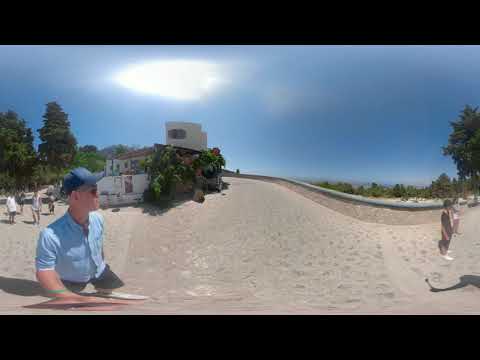This horizontally-aligned, rectangular photograph features a thick black border at the top and bottom. The upper part of the image displays a predominantly cloudy sky, with dark gray clouds obscuring much of the area but opening up to a bright white patch in the upper left. Below, the scene captures a light brown, sandy ground, covered with footprints, suggesting a well-traversed area which might also be paved with cobblestones typical of an arid, desert-like setting.

On the left, a man, possibly of Asian descent, walks towards the right. He is wearing a blue ball cap, sunglasses, and a light blue button-down shirt paired with dark shorts, and his legs appear blurred, adding to a dynamic quality. His right arm, adorned with a green band, is extended, possibly distorting due to camera effects, making it seem as though he's taking a picture. Further in the background on the left, more people are visible, walking in his direction, with a cluster of tall, green trees towering behind them. A multi-story building, potentially an apartment complex, partly obscures from view with foliage in the foreground.

Toward the right side of the photograph, a couple of other individuals stand distantly. One is distinctly clad in black attire with white shoes, while the other’s details are indiscernible. These figures appear to be gazing towards the right side of the frame, positioned near an open courtyard and a low, stone-fenced area. The background on this side also features more trees and brush, emphasizing the outdoor setting. The entire scene is bathed in bright sunlight emanating from a blue sky, creating a midday ambiance. The overall graininess and slight wave effect in the imagery hint at unique camera effects and give the scene an intriguing, vintage feel.